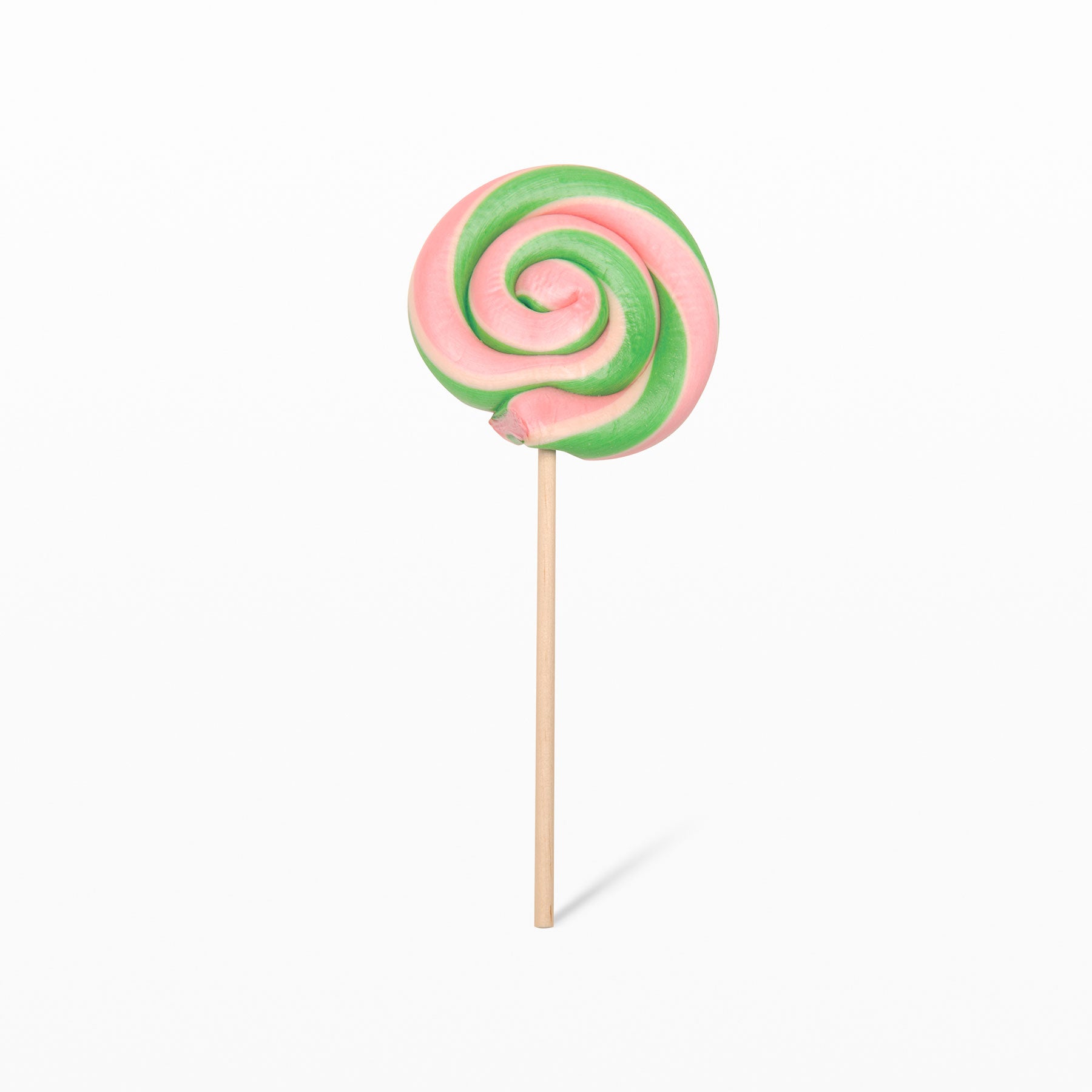This color photograph features a handmade, old-fashioned lollipop prominently centered against a completely white background. The lollipop, characterized by its thick composition, swirls in harmonious, alternating shades of pink and green. It appears to have been crafted from a tube of candy, coiled in a circular, multi-layered spiral formation, evident by the deep crevices where the candy folds over itself. This lollipop, also referred to as an all-day sucker, is secured on a long, pale wooden stick, which casts a faint shadow on the pristine backdrop. The image solely focuses on the lollipop, with no additional elements or writings, capturing its intricate, vibrant swirls with meticulous detail.